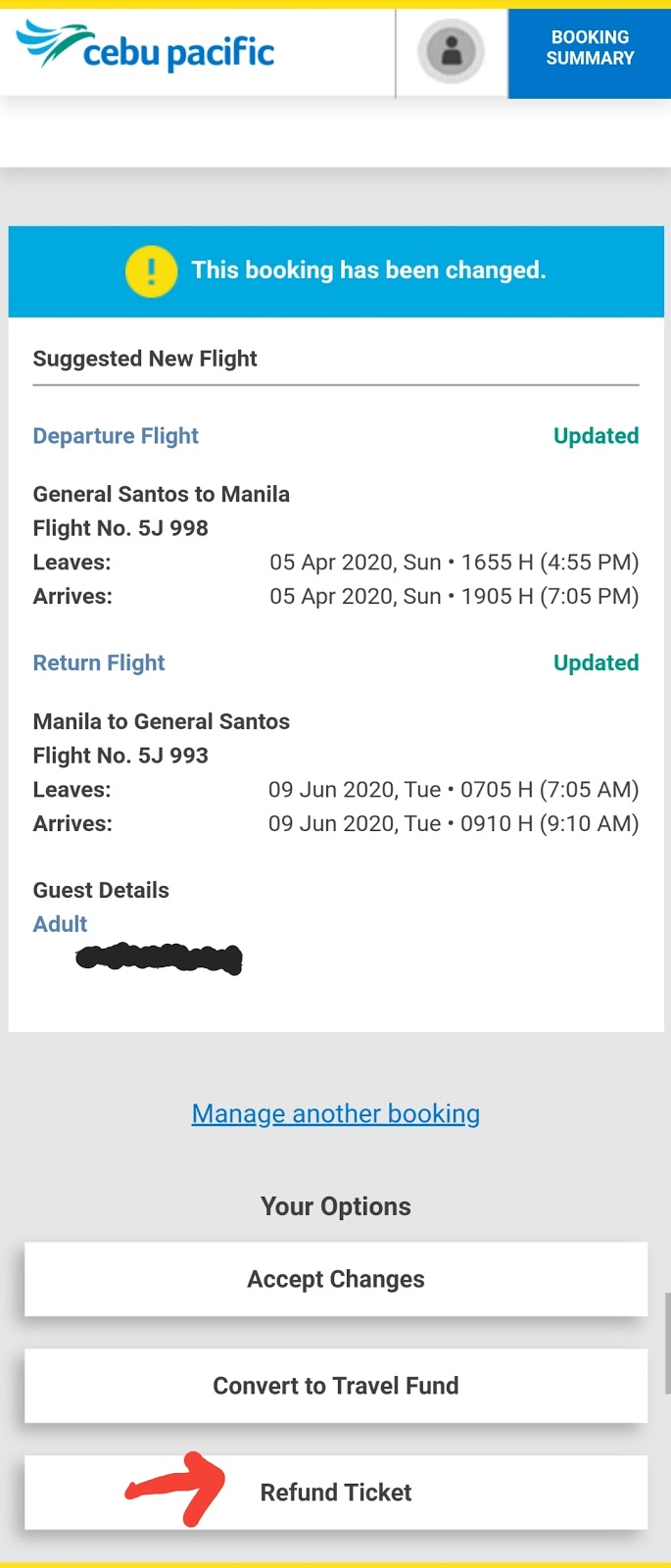At the top of this web page, there is an emblem depicting green and blue waves, next to which is the text "CEBU Pacific" followed by "Booking Summary." Below this header, there is a gray rectangle with no content. Beneath the gray rectangle is a blue one featuring a yellow circle with a green exclamation point inside. The text within the blue rectangle, written in white, states, "This booking has been changed."

Below the blue rectangle, there is a white one that reads "Suggested New Flight" in black ink, with a gray line underneath. To the left, in blue text, it says "Departure Flight," followed by "General Santos to Manila, Flight Number 5J998" in black. This section includes details such as the departure and arrival times. To the right of "Departure Flight," the term "Updated" is written in green.

Further down on the left, "Return Flight" is displayed in blue text, also accompanied by "Updated" on the right. The black text underneath indicates "Manila to General Santos, Flight Number FJ993," alongside the flight's departure, arrival times, and a date: June 9, 2020.

Below this, on the left side, it shows "Guest Details," with "Adult" in blue text that has been scribbled out with a marker. Following this, there is another gray rectangle with "Manage Another Booking" in blue text and "Your Options" in black text centered within the rectangle. Within this section, there are three white buttons: "Accept Changes," "Convert to Travel Fund," and "Refund Ticket." The "Refund Ticket" button is marked with a red arrow drawn with a marker on the left side.